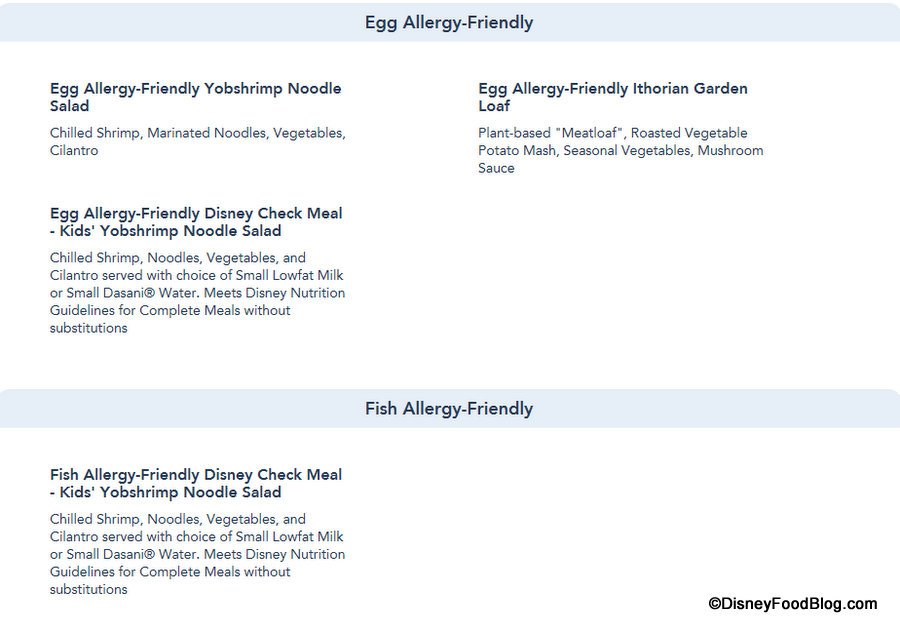**Detailed Caption:**

This image depicts a webpage titled "Egg Allergy Friendly," designed with a blue and white color scheme. At the very top, the title "Egg Allergy Friendly" is prominently displayed in bold black letters. Directly beneath the title, in the first row, the page features the "Egg Allergy Friendly Yop Shrimp Noodle Salad," which consists of chilled shrimp, marinated noodles, various vegetables, and a sprinkle of cilantro.

Additionally, the first row highlights the "Egg Allergy Friendly Arthurian Garden Loaf," a plant-based meatloaf accompanied by roasted vegetables, potato mash, seasonal vegetables, and a savory mushroom sauce.

Moving to the middle of the page, there is a section for kids: "Egg Allergy Friendly Disney Check Meal for Kids Yop Shrimp Noodle Salad." This dish includes chilled shrimp, noodles, vegetables, and cilantro, and is served with a choice of either small low-fat milk or small Dasani water. It adheres to Disney Nutrition Guidelines for complete meals without substitutions.

Finally, at the bottom of the page, another section, labeled in black lettering, presents "Fish Allergy Friendly" options. It again features the "Fish Allergy Friendly Disney Check Meal Kids Yop Shrimp Noodle Salad," with the same ingredients and serving options as the egg-friendly version, ensuring it meets Disney's nutritional guidelines for complete meals without substitutions.

The information and image appear to be sourced from DisneyFoodBlog.com.